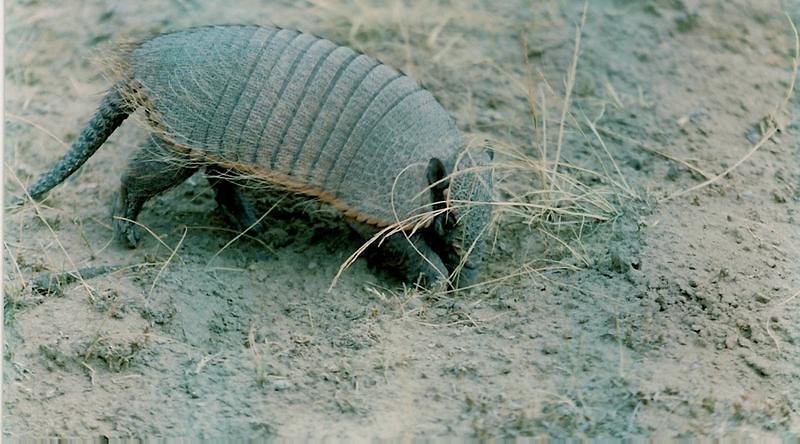The image is a rectangular outdoor photograph set in a desolate, desert-like landscape. The terrain is dry and barren, composed mostly of sand and dirt with sparse patches of scraggly, dead hay-like grass sporadically emerging from the ground. The focal point of the photograph is an armadillo in motion, as evidenced by the positioning of its legs and its forward stride. The armadillo is primarily gray with a touch of pink, accentuated by reddish-brown, wispy hair trimming around its shell. Its tail hangs down and also bears some smaller hairs. The creature’s armor displays distinct lines and ridges, characteristic of an armadillo's protective shell. The animal's coloring allows it to blend subtly with the earthy tones of its surroundings, providing a natural camouflage in the sandy and straw-strewn environment.